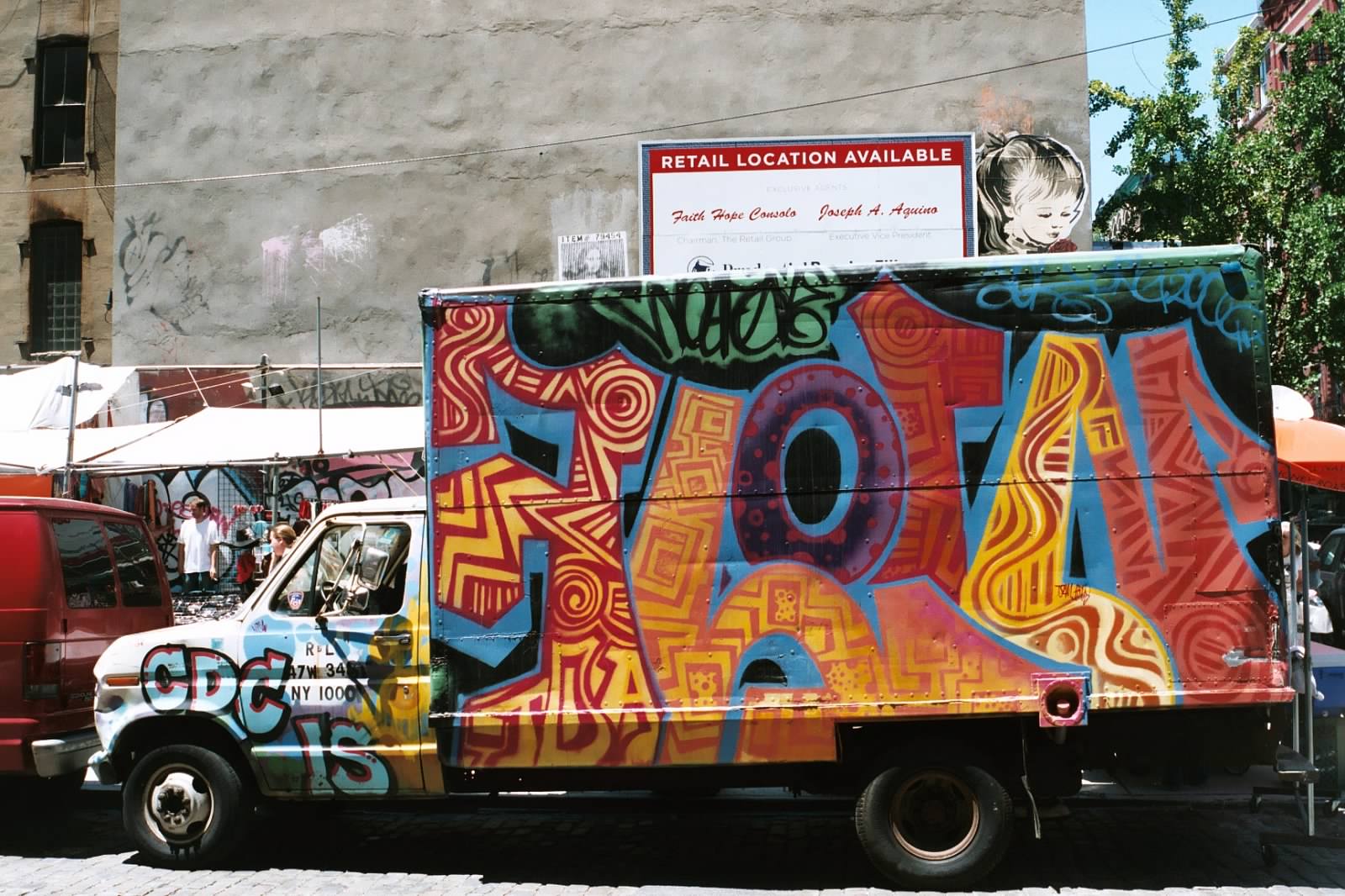The image features a mid-size box truck, adorned with vibrant graffiti and various colors such as red, yellow, blue, and green. The graffiti, essentially a mural, covers the truck's cab and entire side panel, presenting abstract and unreadable designs. Notably, the front of the truck bears the phrase "CDC is." The truck is pointed to the left, and in front of it, the rear end of a red van is visible.

Background elements enhance the scene's complexity. Behind the truck, there's a tall gray building with a wall that lacks visible windows or doors. A poster on the building advertises a "retail location available," and next to this poster, there’s an image of a girl's face. Adjacent to this building, on the right, stands a tall green tree, partially concealing a red brick building with its lush foliage.

At the lower left side of the image, several people can be seen gathered beside a tent, indicative of a local event or market. They appear to be situated between the red van and the truck, emphasizing the scene's bustling urban atmosphere.